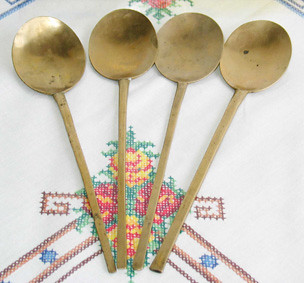This photograph features four brassy gold spoons with long, straight handles and circular, semi-flat bowls. The spoons are neatly arranged on an embroidered white fabric that resembles a tablecloth. The intricate embroidery features a cross-stitch pattern forming corner points with vibrant roses in hues of red, yellow, and orange, surrounded by green leaves. Additional colors in the embroidery include browns, blues, and pinks, contributing to the floral and geometric design. The spoons are aligned with their large, circular bowls at the top of the image and their slender, flat-ended handles converging towards the bottom, creating a harmonious and detailed composition.